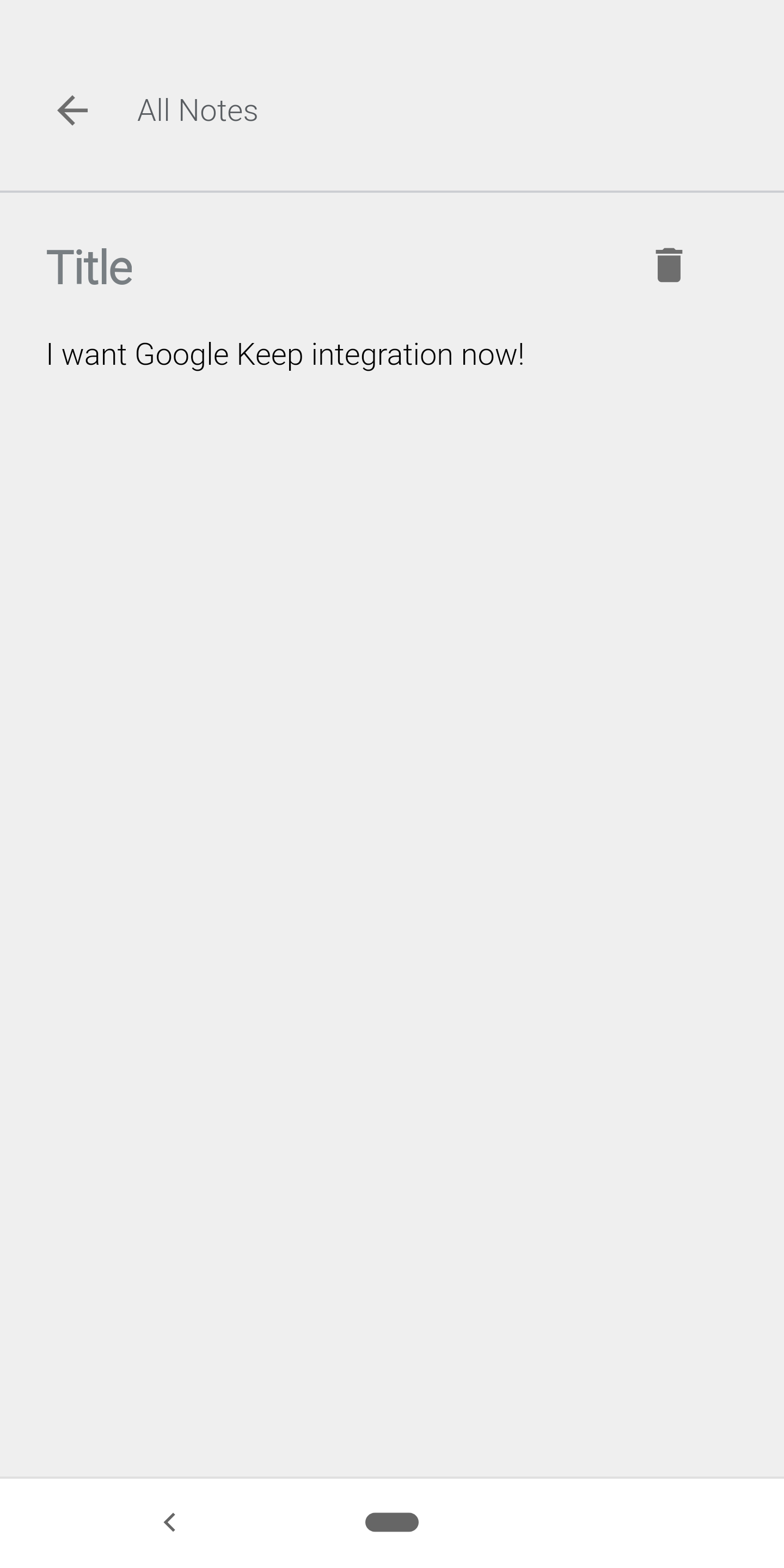The image appears to be a screenshot taken from a smartphone, characterized by its rectangular shape that is approximately three times longer than it is wide. The background is a light grayish color. Positioned around two inches from the top is a darker gray horizontal line. Above this line, there's a black arrow pointing to the left, and to its right, the text "All Notes" is written in black with both 'A' and 'N' capitalized.

Below the darker gray line, on the left side, the word "Title" is displayed in larger black lettering. On the right side, there's a black trash can icon, likely representing a delete option. 

Under the "Title" text is a slightly smaller phrase in black that reads: "I want Google Keep Integration!," emphasizing 'Google' and 'Keep' with capital G and K, respectively, and ending with an exclamation point. The area beneath this text is blank, extending down to the bottom where there is an about one-inch wide white strip.

On the left side of this white strip, approximately an inch from the edge, there is a black greater than symbol (>) pointing to the left. Near the center, if you measure about a quarter inch to the left and right, you find a gray block near the top, repeating the text "All Notes" with 'A' and 'N' capitalized. This description captures the essence and details of the screenshot.